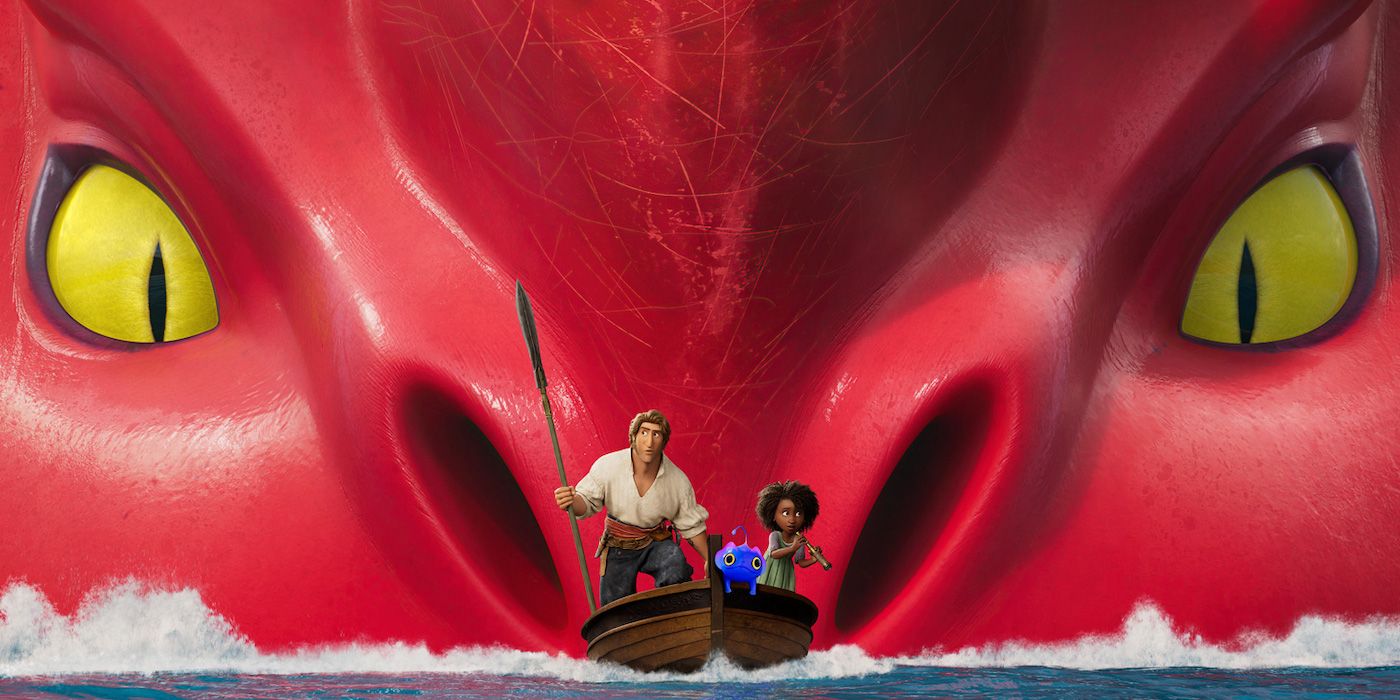The image depicts a detailed scene from a 3D animated movie, possibly resembling a Disney or How to Train Your Dragon style film. Dominating the background is a massive red sea dragon, distinguished by its striking yellow, snake-like slit eyes and black pupils. The dragon's nostrils are prominently red, enhancing its fierce appearance. In the foreground, there is a wooden boat navigating through choppy, white-capped waves. Onboard the boat is a man with brown hair, wearing a white shirt and blue jeans, holding a spear. Accompanying him is a young Samoan or black girl with curly black hair, who appears to be holding a telescope. Additionally, a small blue creature with an antenna is present, adding a whimsical touch to the scene. The intricate details and vibrant colors make the image visually compelling and rich in narrative elements.